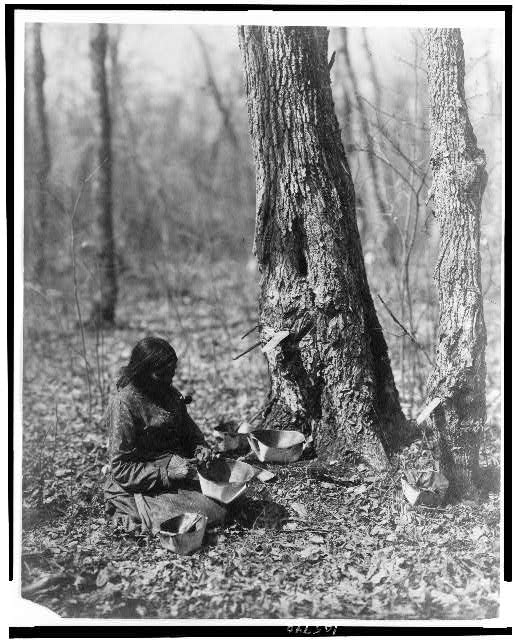This historic black-and-white photograph, set in a stark, leafless forest that appears either dead or burned-out, depicts a woman of possible native background sitting cross-legged on the forest floor. The scene features a densely wooded area with crinkled leaves scattered on the ground and several trees, including one with visible holes and a device protruding from its trunk, suggesting sap extraction, likely for maple syrup. The woman, with dark hair and dressed in heavy, primitive attire including a long-sleeved dress and apron, is focused on her task, which involves handling three metal pots positioned around her—one in her lap, another by her side, and the third near a tree. She appears to be transferring something, possibly sap or mushrooms, from a stick into the pots. The aged photo, bordered in a black frame with worn corners, contains some indistinct text at the bottom, enhancing its historic nature.